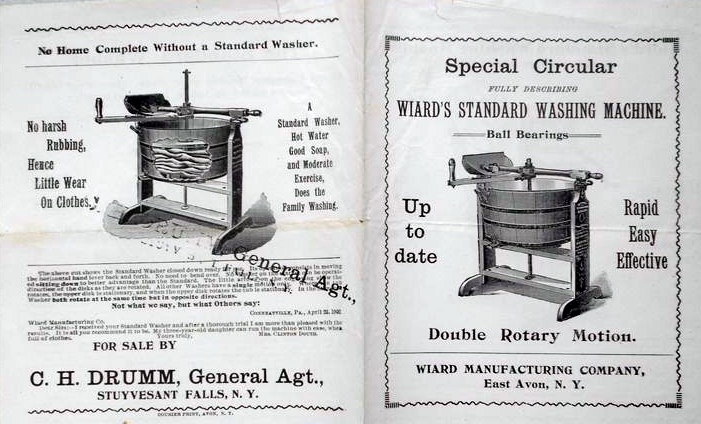This image is a vintage advertisement from the early 20th century, likely sourced from an old newspaper or magazine. The ad is for a hand-crank washing machine, prominently featuring the slogan, "No home complete without a standard washer." It highlights the benefits of this non-electric washer, including "no harsh rubbing, hence little wear on clothes" and its efficacy when combined with "hot water, good soap, and moderate exercise" to handle the family's washing. The advertisement details key features of the machine, including "ball bearings," "up-to-date, rapid, easy, effective double rotary motion," and is produced by the Wired Manufacturing Company, East Avon, New York. There is a general stamp indicating it is "For Sale by CH Drum, General Agent, Stuyvesant Falls, New York." The left side of the ad emphasizes customer testimonials with the phrase, "Not what we say, but what others say." The advertisement is presented in black and white with basic fonts, capturing the simplicity and practicality of early 20th-century marketing.